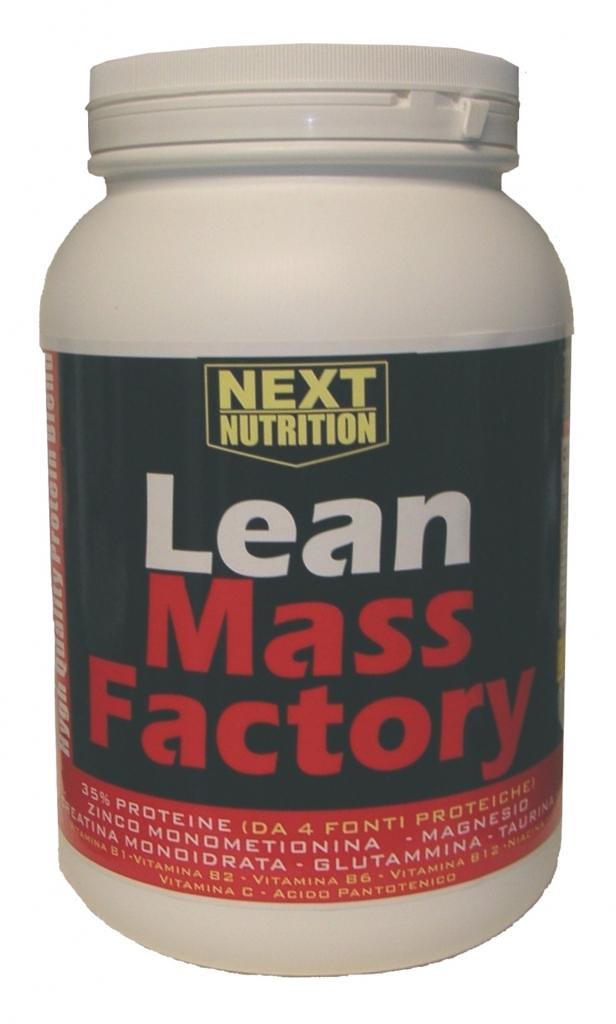The image features a white plastic container with a matching white top. The top appears to be sealed, indicated by a strip along the bottom ridge that will break upon first opening. The design includes a noticeable ridge around the lid for better grip. The container itself has a jar-like shape and is adorned with a dark, possibly black, label that is bordered at the bottom with a red stripe. 

Prominently displayed on the label, in gold or yellow letters, are the words "Next Nutrition" inside a downward arrow-shaped box. Directly below, the word "Lean" is written in white letters, followed by "Mass Factory" in red letters. 

Additional details are provided in the red-bordered section at the bottom of the label, which highlights that the product contains 35% protein. The label also features more comprehensive information about the ingredients, including vitamins, and possibly some text in different languages, which might be difficult to recognize without translation.